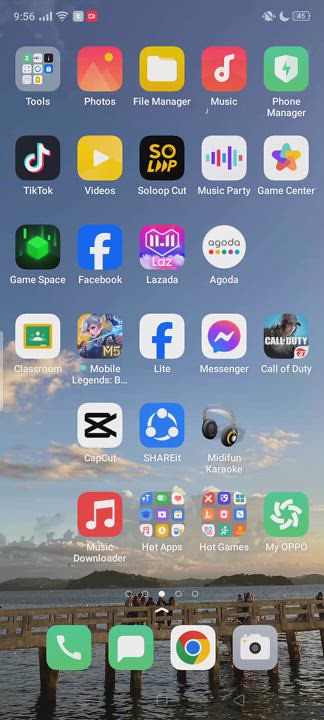This screenshot from a mobile smartphone captures its home screen adorned with a picturesque background image. The photograph features a concrete bridge stretching over a vast expanse of water, supported by round concrete pylons. A few individuals are seen standing on the bridge, peering over its edge into the water below. In the background, a series of tree-covered low-lying islands are visible under a sky painted in hues of light blue and dark grey with scattered clouds.

Superimposed on this scenic background is a grid of app icons organized neatly, indicative of a typical smartphone home screen layout. At the top of the screen, the status bar displays essential information: the current time, cellular signal strength, Wi-Fi connection status, two additional icons, and the battery level, which shows at 45%. Additionally, the 'Do Not Disturb' mode is active, as indicated by its corresponding icon.